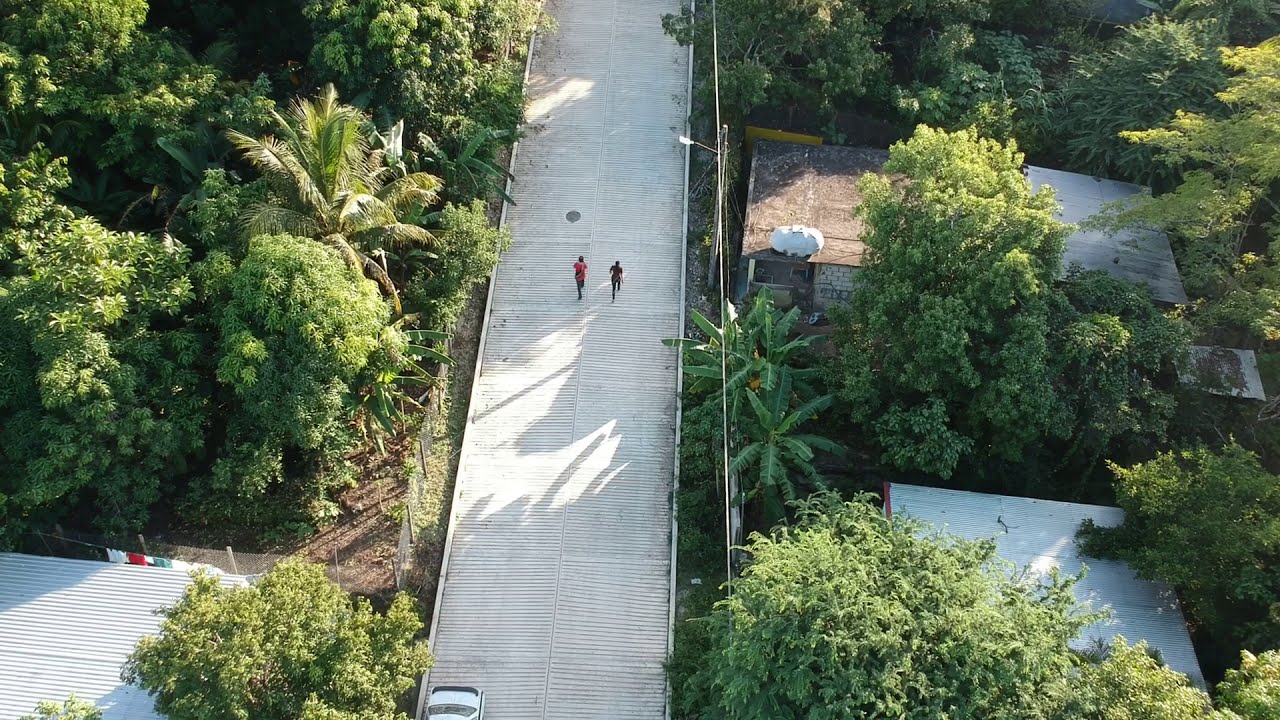A vibrant scene depicts a narrow, slotted metal bridge extending through a lush, green, and sunny landscape. The bridge, appearing white or silver in color, supports two lanes of traffic. Two people, one wearing a red shirt and the other in black, are jogging right down the middle of this bridge, with a car following not far behind. On either side of the bridge, dense clusters of trees, including several palm trees, frame the view. Both sides are flanked by green foliage and various rooftops, with some buildings showing white and brown colors. On the left side, a structure with a clothing line displays garments in white, red, blue, and green. The right side also reveals more housing structures, adding subtle architectural elements to the picturesque outdoor setting.